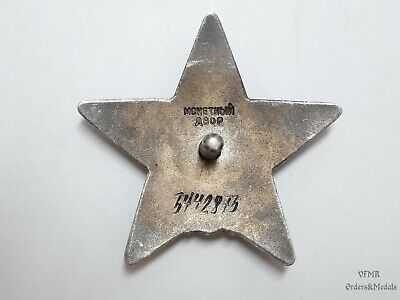The image features a vintage, star-shaped medallion or badge resting on a featureless white or gray surface, casting slight shadows around its edges. The star, which could possibly be a sheriff's badge, is metallic and shows signs of discoloration on its back, indicating age and wear. A central circular protrusion, rather than a pin, is visible, likely for affixing the badge to clothing. Stamped text above this protrusion is difficult to decipher, although various attempts suggest it could say "M-O-M-G-T" or similar. Another set of stamped text and symbols follows below, potentially reading "B-O-P", with "Bureau of Police" as one possible interpretation. At the bottom of the badge, a long number, 3442843, is inscribed in black ink, possibly indicating a serial number. The bottom right of the image features a watermark that reads "VFMR Orders and Medals." The back of the badge also shows additional stamped text that is mostly unreadable due to its ingrained nature.